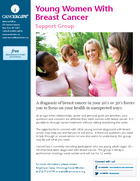This pixelated image appears to be a flyer for a support group. The title, prominently displayed in pink, reads "Young Women with Breast Cancer." Beneath, in smaller text, is the phrase "Support Group." The central image shows four women smiling warmly at each other, standing outdoors in a park or wooded area. They are closely huddled, with their arms draped around each other's backs, forming a circle. 

Around the edges of the flyer, there are additional details, although the resolution makes it challenging to decipher. On the right-hand side of the flyer, a table with three unreadable rows presents multiple options or pieces of information. The left-hand sidebar includes a banner that likely details the organization or company hosting the support group, along with possible contact information or other services. There also appears to be a blue button indicating something available for free, although the exact nature of this offering is unclear. At the bottom of the flyer is a partial phone number, suggesting a hotline or direct contact for support.

Overall, the flyer aims to provide essential information about a support group for young women with breast cancer, emphasizing community and mutual support with the imagery of women united in solidarity.